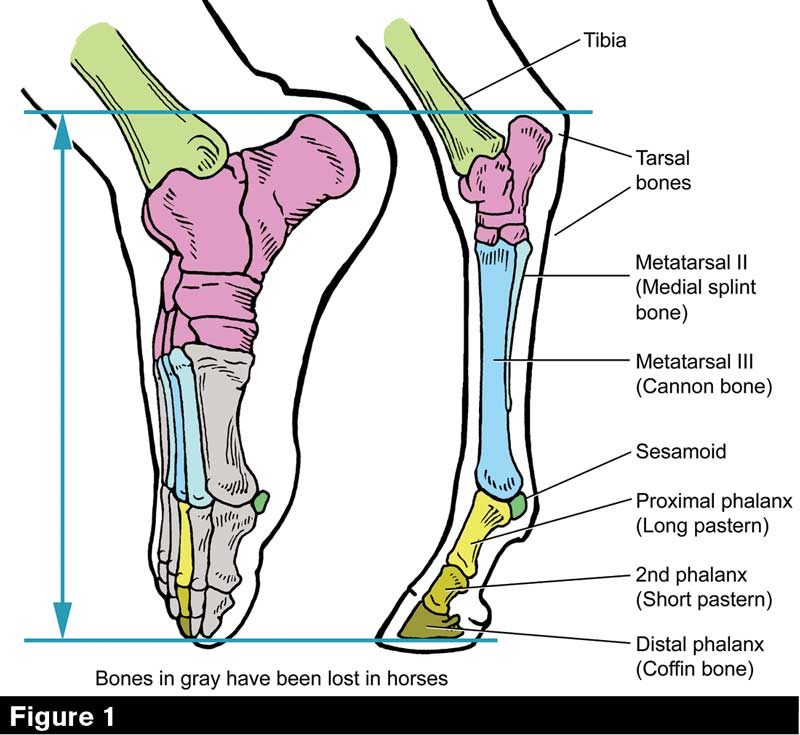The image is an infographic labeled "Figure 1," illustrating a comparative anatomy of a human foot and a horse's hoof. On the left side, it depicts the human foot, and on the right, the horse's hoof. Each bone is distinctly colored to show their counterparts in both species. The infographic highlights the tibia in green, tarsal bones in pink, metatarsals in cyan, metatarsal 3 in blue, proximal phalanx in yellow, second phalanx in golden yellow, and distal phalanx in green. It also notes that bones shaded in gray represent those that have been lost in horses through evolution, revealing significant structural similarities between human feet and horse hooves. The diagram effectively educates on the skeletal transformation and comparative anatomy, emphasizing that horses have evolved by losing several toes, making their hoof structurally analogous to the human foot in several aspects.